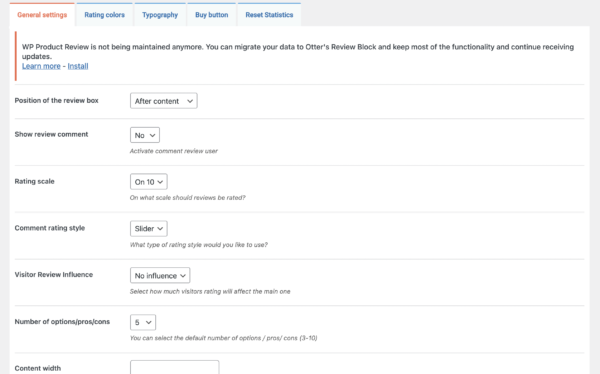The image depicts a settings page with a clean, all-white background. At the top left, four hyperlinked boxes are displayed in blue text, reading from left to right: "Rating Colors," "Typography," "Buy Button," and "Reset Statistics." The first box, "General Settings," highlighted in orange text, indicates the current selection.

Beneath these options, there is a notification bar that reads: "WP Product Review is not being maintained anymore. Migrate your data to other review blocks to keep most functionalities and continue receiving updates." Following this message, there are hyperlinked texts "Learn More" and "Install" in blue with underlines, accompanied by a vertical orange bar to the left.

Further down, a series of module selection boxes detail various settings. The first box, titled "Position," has "Position the Review Box" with the option "After Content" selected. Below, "Share Review Comments" is marked with the selection "Not a Third-Party Review User." The "Rating Scale" is set to 10, and the "Comment Rating Scale Slider" follows. Below that, "Visitor Reviewer Influence" is marked with "No Influence" selected. The "Number of Options" is set to five. The final module, "Content Width," is presented with an empty text box.

This detailed layout suggests user customization options for a review plugin, emphasizing the positioning and interaction metrics for user reviews.